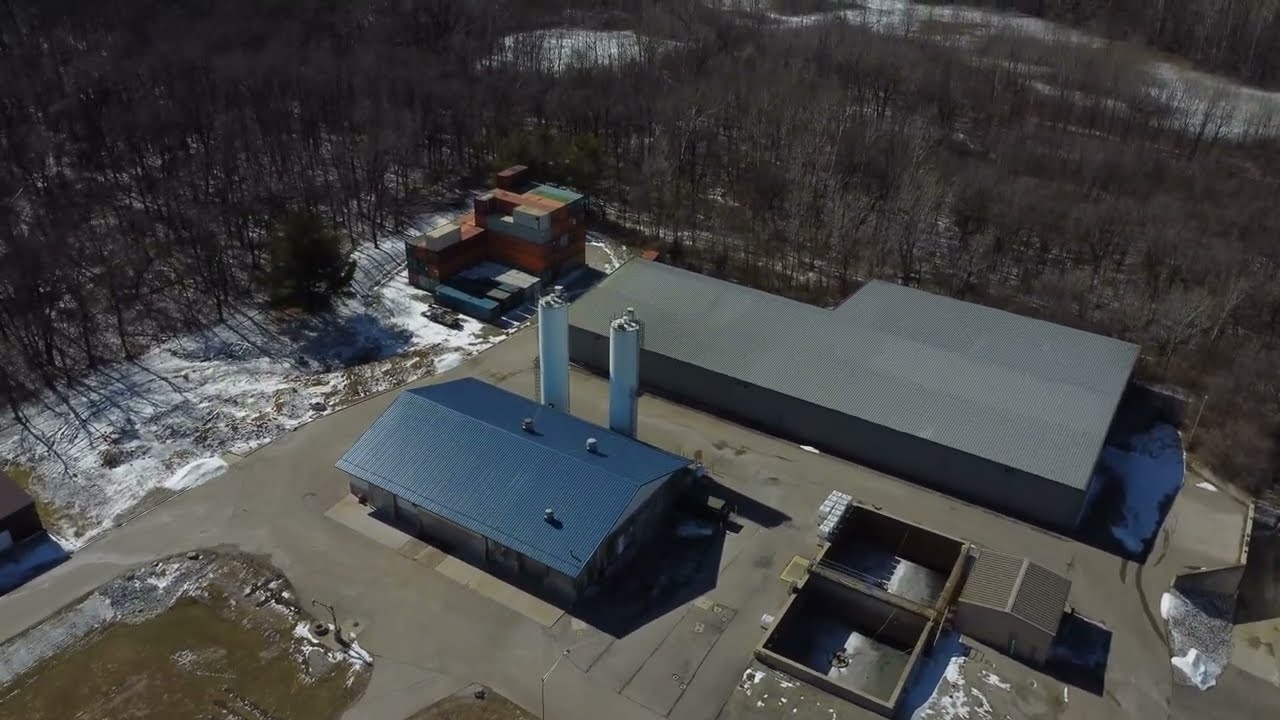The image depicts an aerial view, potentially captured by a drone, of an industrial area carved out in the middle of a dormant, winter forest. Central to the scene is a single-story building with a dark blue metal roof, adjacent to which stand two tall, narrow light blue tanks. On the opposite side of the tanks lies a much larger building, uniformly gray with a matching roof and walls. In the upper left section of this larger building, multiple storage containers in assorted colors—red, white, blue, and black—are stacked on top of each other. These containers are positioned slightly away from the main concrete area, surrounded by a light dusting of snow. The ground below presents a mix of tan and gray hues, sporadically covered with snow. The background is dense with leafless trees, their barren branches adding to the scene’s wintry atmosphere, with sporadic patches of snow visible among them. Overall, the setting is clearly outdoors, encompassed by a forest, and gives the impression of being part of a factory or business compound in a cold, wooded area.